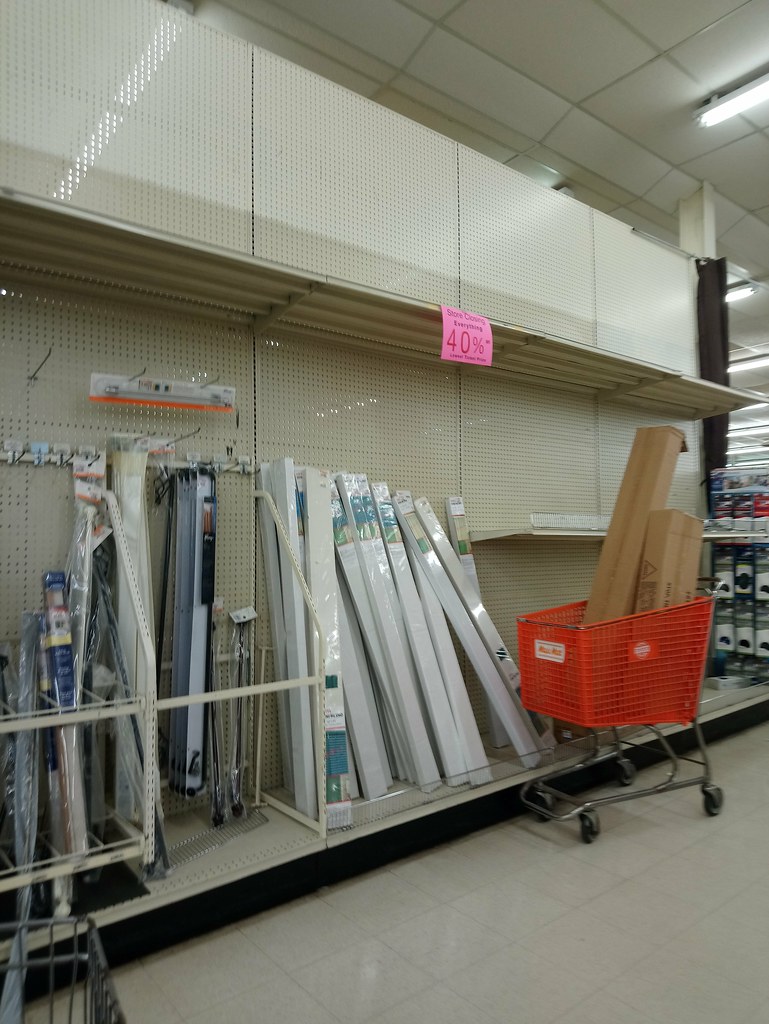In this color photograph of a store, the focus is on a single row of shelves against a backdrop of off-white, beige floor tiles arranged in a square pattern. Visible in the lower right corner is part of the tiled floor. A red shopping cart is situated slightly further up to the right. Two long, thin boxes are protruding from the back of the cart. 

The top shelf of this section is completely empty, but prominently displays a "40% off" sign. The middle shelves are stocked with long, thin white items, grouped centrally. To the left of these items, there are additional products leaning against the shelf, although their details are indistinct. In the background, to the far right, another shelf can be partially seen, filled with a variety of items that are not clearly discernible.